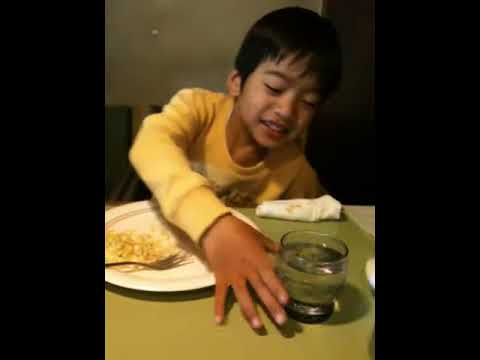In the image, a young boy with black hair and light caramel skin, wearing a yellow long-sleeve shirt, is captured in a moment of joy with a subtle smile on his face and his eyes slightly closed. He is seated at a lime green table over which he is reaching with his right hand towards a small, transparent glass, most likely filled with water, placed at the bottom right corner of the table. The boy's left hand is not visible, suggesting it might be under the table. Nearby, a neatly folded white napkin rests close to him. Positioned to the left of the glass is a white plate with a distinct reddish-orange rim, holding what seems to be a yellow-colored food item, possibly a fried egg, along with a silver fork. The table scene is set against a cream or gray colored wall, with the boy sitting on a dark colored chair. The image also has black borders on the left and right sides, indicating it might be a screen capture, possibly from a smartphone. The overall composition suggests an everyday moment, perhaps captured in a kitchen setting.